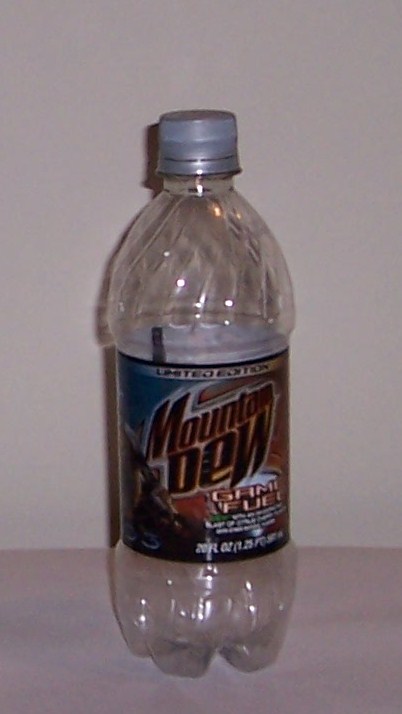This photograph showcases an empty Mountain Dew bottle placed on a white surface, possibly a countertop or floor, with a white wall in the background. The bottle is entirely devoid of liquid and features a silver cap. The bottle itself is mostly translucent with a slight opaqueness. Positioned centrally in the image, the bottle's label prominently displays the Mountain Dew logo in bold black text, accentuated with a reddish-orange hue between the letters and bordered by white. The font used for the logo has an energetic, action-packed style. In the bottom left-hand corner of the label, a character can be seen, adding to the dynamic theme. Additionally, the label indicates "Game Fuel" and specifies just below the top that this is a limited edition version of the drink. The overall composition is centered and clear, capturing the distinctive details of the label and the bottle.